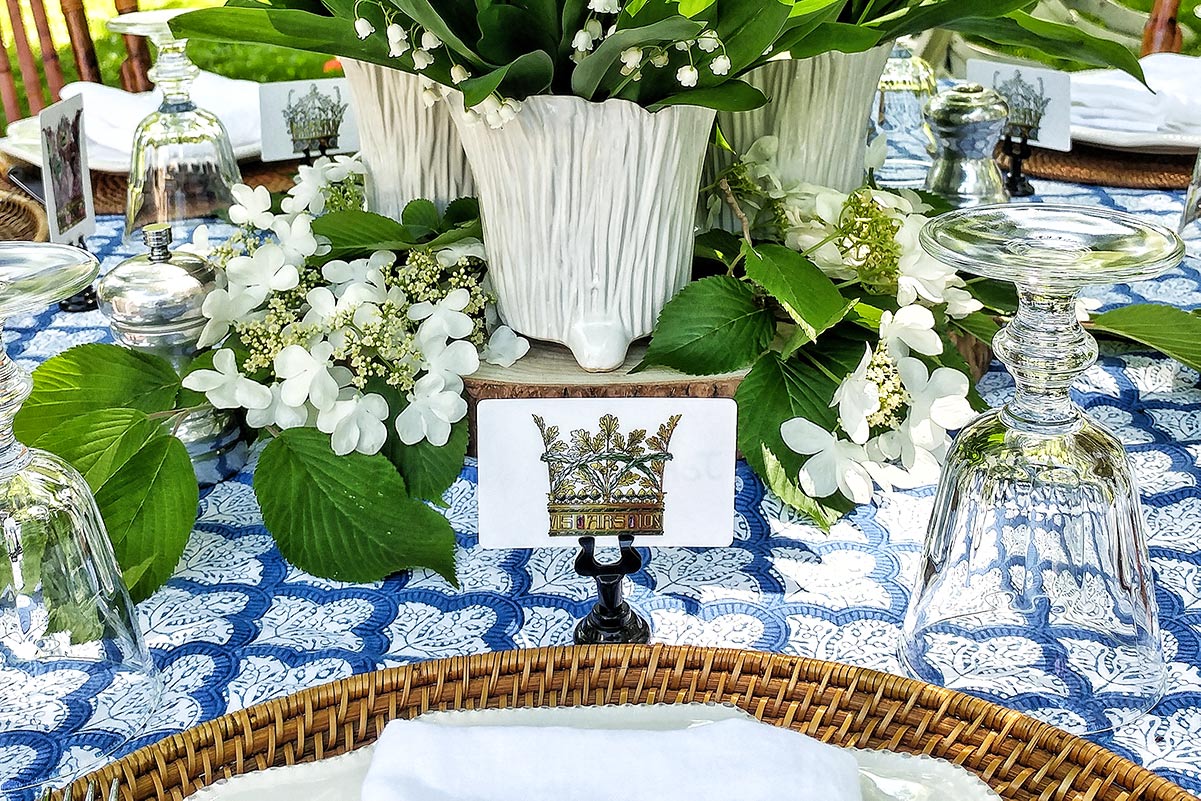The color photograph is a detailed close-up of an elegantly set table adorned with a blue and white diamond patterned tablecloth. At the heart of the table is a centerpiece featuring delicate lily of the valley flowers in white ceramic containers, surrounded by green leaves. A decorative woven basket sits prominently in the foreground, and placed nearby is a card holder displaying a card with a golden crown, inscribed with "B-I-S-A-R-S-I-O-N." Crystal goblets are meticulously arranged around the table, all turned upside down, suggesting a formal or special event. The bright daylight enhances the festive atmosphere, revealing additional table settings in the background and casting a natural glow over the scene.